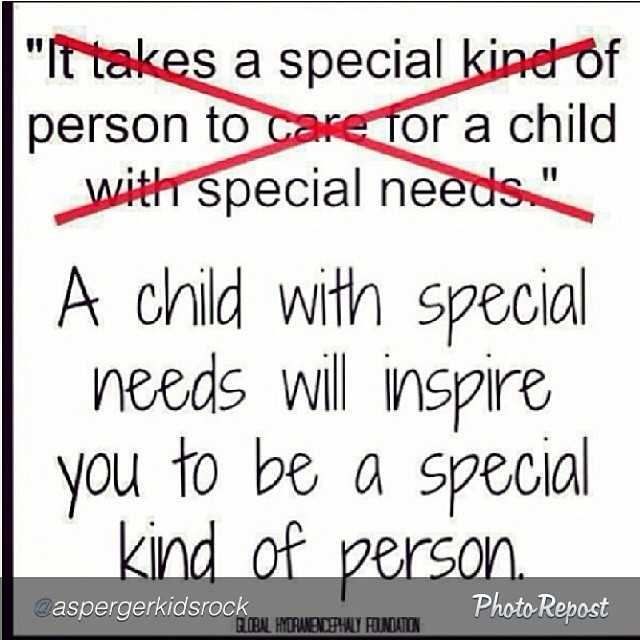The image is a digitally created poster on a white background, framed with thin black lines and featuring red, gray, and black tones. The top section of the poster displays a quote, "It takes a special kind of person to care for a child with special needs," which is manually crossed out with a bold red X. Beneath this, written in a black handwriting font, is the revised message: "A child with special needs will inspire you to be a special kind of person." At the bottom of the poster, there is an overlay text stating "At Asperger Kids Rock Photo Repost," with the additional notation "Global Hydroencephaly Foundation" present in the description.